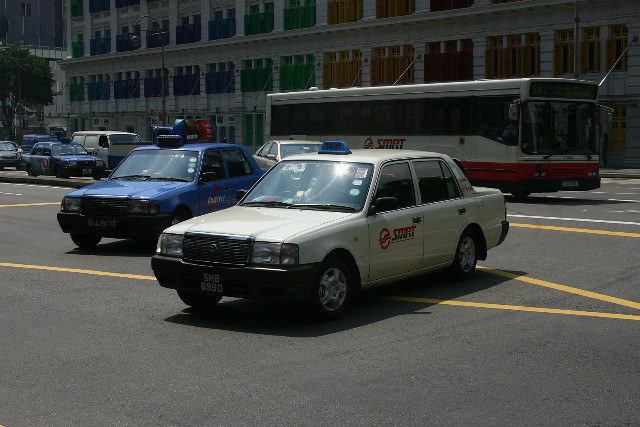The photograph, taken in landscape orientation and natural daylight, showcases an urban scene dominated by two cars at the forefront. In the center, a large grey saloon car, possibly a taxi given the blue sign on its roof and the red writing on its left door, faces slightly to the left. The sun casts a bright reflection on its windscreen. To the left and slightly behind is another vehicle, a blue four-door sedan, which also bears a sign on its roof. The grey tarmac surface below the cars is marked by yellow lines, indicating traffic guidance.

Behind the saloon cars, a white and red city bus is visible, sporting a grey top and red trim along its bottom edge. The bus is positioned on a road also marked by white lines. Further into the background, a white van and another blue car can be seen, completing the busy street scene.

The backdrop of this bustling area is a very long, multi-floored building extending from right to left, with greyish ornate square windows adorned with bars of various colors: blue, green, yellow, red, and transitioning to darker hues. The upper left-hand corner of the image features trees along the building's edge, adding a touch of greenery to the urban landscape.